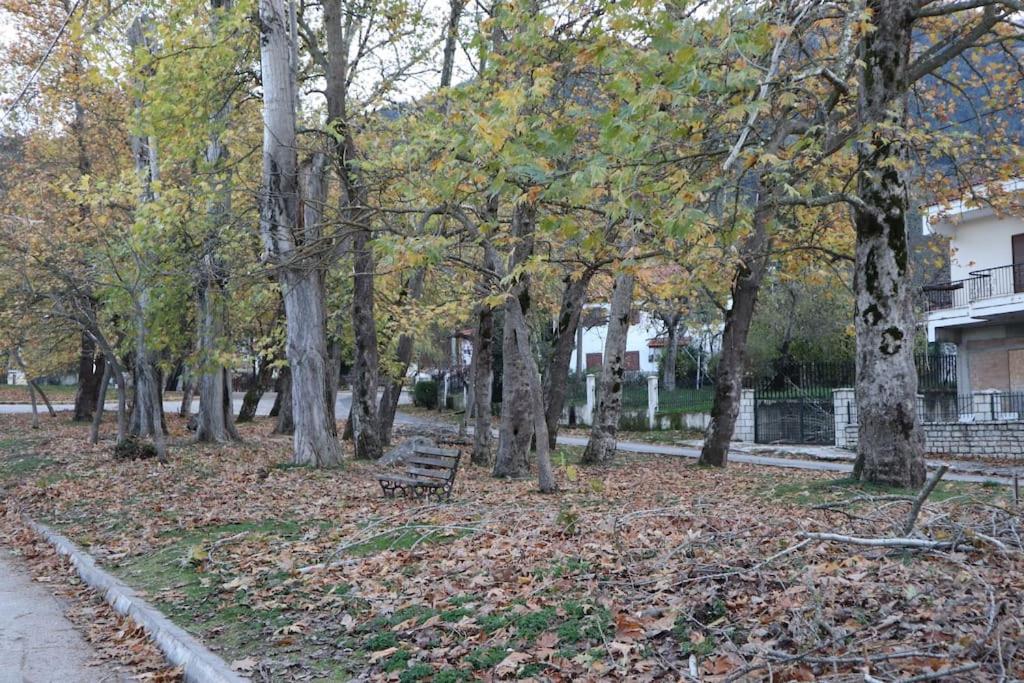This horizontal rectangular photograph captures a vibrant autumn scene of a divided street featuring a central park-like island. The focal point is the tree-lined grassy median, scattered with numerous fallen brown leaves and interspersed with around ten large tree trunks, primarily gray with some black markings. Among the trees stands a solitary wooden park bench, inviting passers-by to pause and enjoy the surroundings. To the right side of the image, a row of houses or apartment buildings can be seen, characterized by white structures with windows and black fencing, demarcating their front yards. Beyond the central divider runs a road, while a small portion of pavement and a curb is visible on the left side. This photograph distinctly captures the seasonal essence of fall with an abundance of leaves covering the ground and branches still holding on to some green and colored leaves.